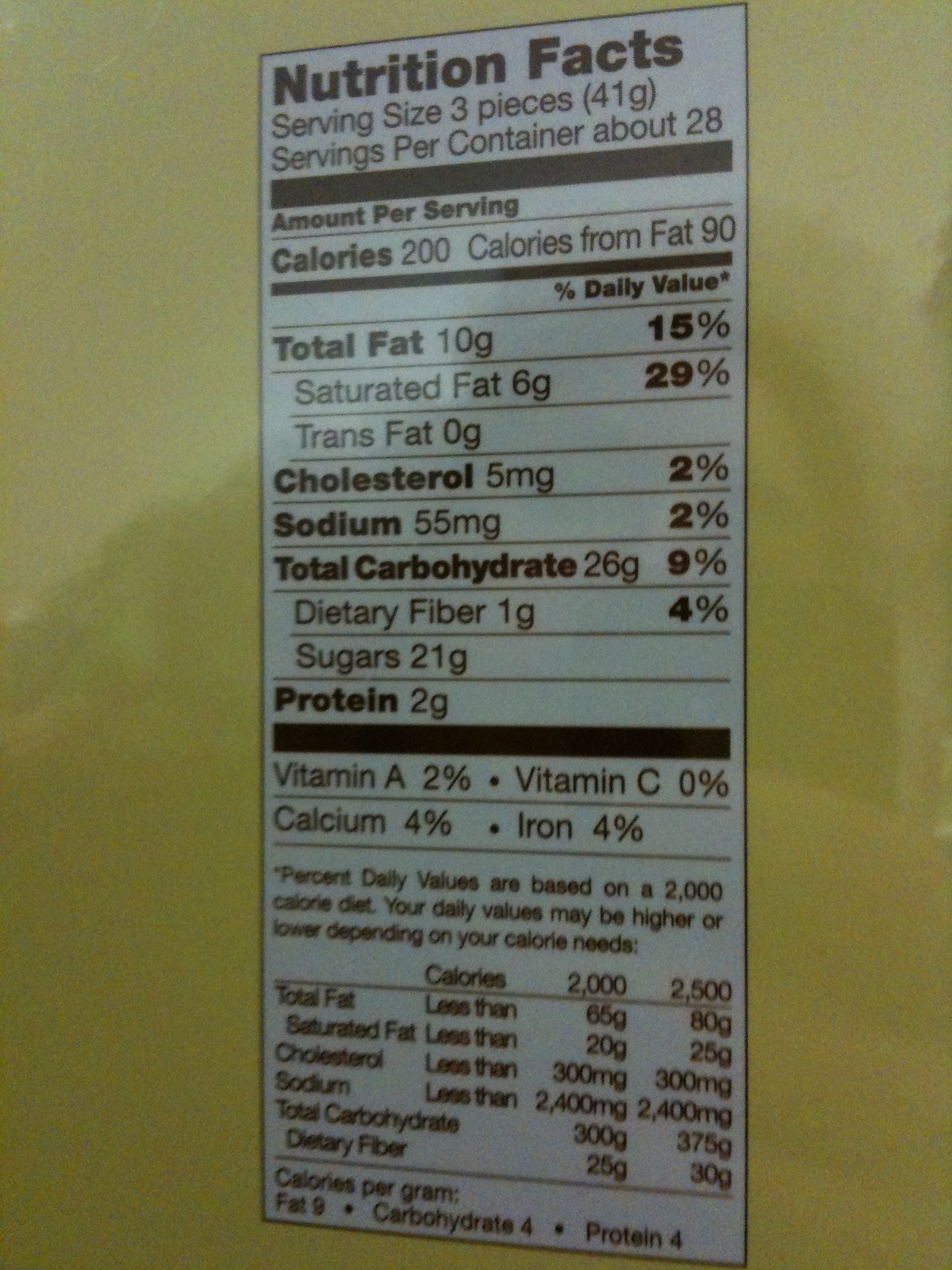This image showcases the nutritional facts label of a product with a yellow background. At the very top, within a white box, the heading "Nutritional Facts" is boldly printed in black and red letters. Below the heading, it details that the serving size is 3 pieces (41 grams), and there are approximately 28 servings per container.

The nutritional breakdown is as follows:
- Calories: 200 (with 80 calories sourced from fat)
- Total Fat: 10 grams
- Saturated Fat: 6 grams (constituting 29% of the daily recommended value)
- Cholesterol: 5 milligrams
- Sodium: 55 milligrams
- Total Carbohydrates: 26 grams

Furthermore, the label provides a percentage of daily values for specific nutrients:
- Vitamin A: 2%
- Vitamin C: 0%
- Calcium: 4%
- Iron: 4%

This detailed information helps consumers make informed dietary choices based on their nutritional needs.